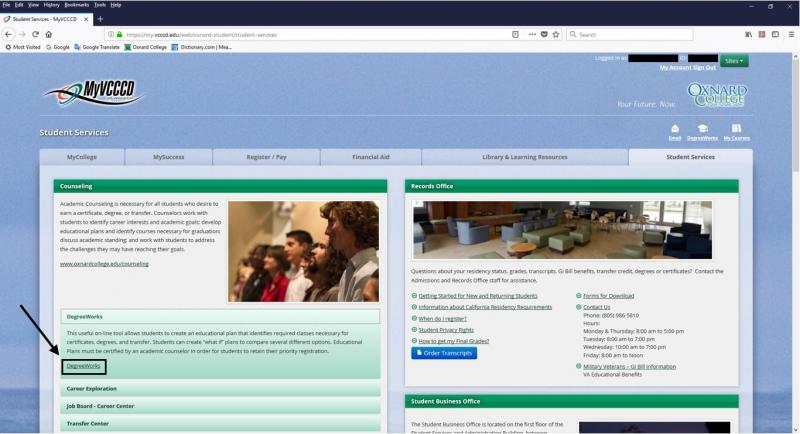This is a detailed screenshot of a website, featuring an educational institution. The background is blue, with the institution's acronym "MYVCCO" prominently displayed at the top left, while the top right corner boldly states "Your Future Now, Oxnard College."

A comprehensive menu bar stretches across the upper portion of the screen, listing several options: "Student Services," "My College," "My Success," "Register/Pay," "Financial Aid," "Library and Learning Resources," and the currently selected "Student Services."

A vibrant green banner marks the section on "Counseling," emphasizing the necessity of academic counseling for students aiming for certificates, degrees, or transfers. This section elaborates on the role of counselors in helping students identify career interests, academic goals, and develop educational plans. It also highlights the importance of addressing academic standing and overcoming challenges to achieve these goals. Adjacent to this text, a photograph depicts several people standing and looking to the left, adding a human element to the information provided.

Another green section titled "Degree Works" outlines a valuable online tool for students to create educational plans. It mentions the capability to draft "what-if" plans for various academic scenarios and stresses the need for these plans to be certified by an academic counselor to maintain priority registration. A hyperlink labeled "Degree Works" is visually emphasized with a black square and arrow.

Beneath this, categories such as "Career Exploration," "Job Board," "Career Center," and "Transfer Center" are listed, although this text appears slightly less defined.

To the right, another green banner labeled "Records Office" appears. It includes a photo of a spacious room filled with tables, chairs, and couches. This section provides information on residency status, grades, transcripts, transfer credits, degrees, or certificates, and directs students to contact the Admissions and Records Office for assistance. It also lists various student-related concerns including registration times, privacy rights, final grades, transcript orders, and accessible forms. Contact details are provided: phone number 805-986-5810, and office hours across the week.

Finally, there is a scarcely visible green banner at the bottom labeled "Student Business Office," indicating the location is "on the first floor of the..." though the rest of the text is cut off in the image.